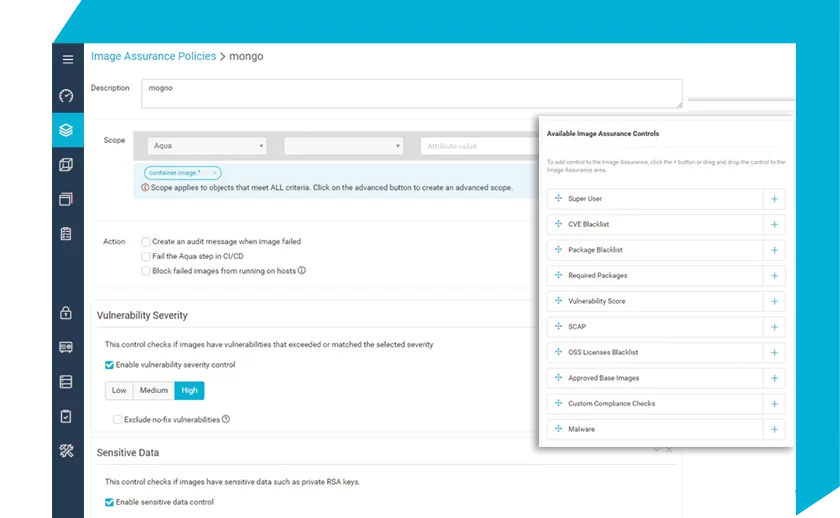This image captures a computer screen displaying a webpage titled "Image Assurance Policies.” At the top of the screen, there is a teal-colored strip that extends horizontally and vertically down the right side, serving a decorative purpose. Below this strip, a row of five icons on the left is visible, housed within a black vertical sidebar. The first icon has been clicked, leading to the current page view, and this icon resembles three stacked papers.

In the header, the text "Image Assurance Policies" is prominently displayed, followed by a right-pointing arrow and the word "Mongo." Further down, a single-line text box labeled "Mongo" has been populated.

The main content area includes various interactive elements for input. These include text boxes for fields like "Scope" and "Action." Additionally, there is a section for "Vulnerability Severity," where the "High" option has been selected, indicated by a teal highlight. Users could also choose "Low" or "Medium" options, although these are currently unselected.